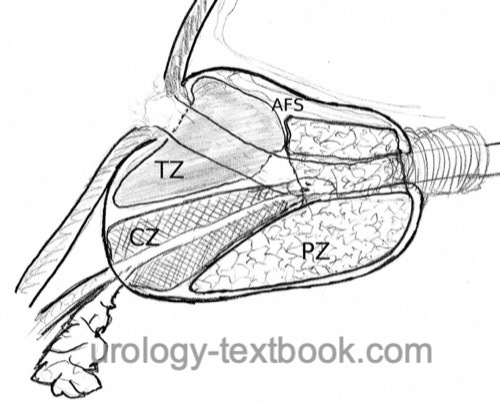This black-and-white image appears to be a detailed pencil sketch of a heart. It features several delineated sections labeled with the abbreviations "PZ," "CZ," "TZ," and "AFS." The sketch shows what looks like various tubes or vessels entering and exiting different regions, indicative of blood flow or structural pathways within the heart. The image includes a watermark that reads "urology-textbook.com," suggesting its source from an educational context. The intricate and meticulous drawing captures the anatomical complexity of the heart, presenting a meticulous representation in a monochromatic style.